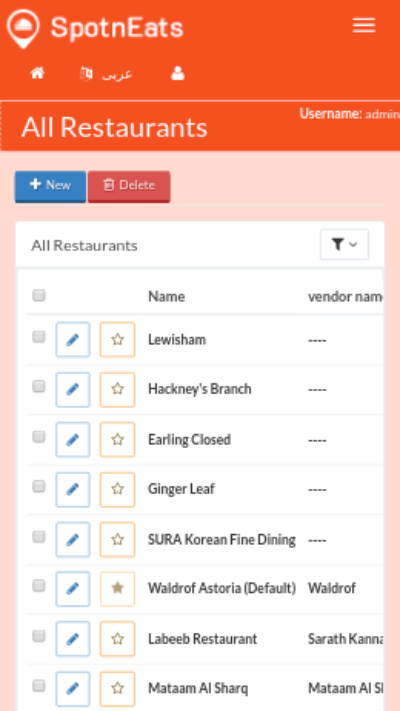In the top-left corner of the interface, labeled "Spot & Eats," the name is spelled out as S-P-O-T-N-E-A-T-S. On the upper right, there are three stacked bars indicating a menu button that, when clicked, displays additional options. Directly below, there is a row of icons: from left to right, a home icon, a calendar icon, and a profile icon representing user settings, all set against an orange background with white text.

Just beneath this section, the text "All Restaurants" is prominently displayed. To the right, the label "Username Admin" is visible, denoting the user’s role. The following section features a peach-colored background, containing two prominent buttons on the upper right corner: a blue "New" button with a plus sign and a red "Delete" button featuring a garbage can icon—both have white text.

Underneath, a white rectangular section displays the text "All Restaurants." To its right is a filter icon accompanied by a drop-down menu for sorting options. Along the left side, there are alternating gray and white boxes with blue outlines, marked with a pencil icon for editing. One box with an orange outline contains a star icon.

The table headers include columns labeled "Box," "Name," and "Vendor Name". The table lists eight restaurant entries as follows:
1. **Name:** Lewis Ham | **Vendor:** (none)
2. **Name:** Hackney Branch | **Vendor:** (none)
3. **Name:** Earl's Closed | **Vendor:** (none)
4. **Name:** Ginger Leaf | **Vendor:** (none)

The description provides a comprehensive overview of the interface layout and button functionalities, ensuring clarity and ease of understanding for the user.